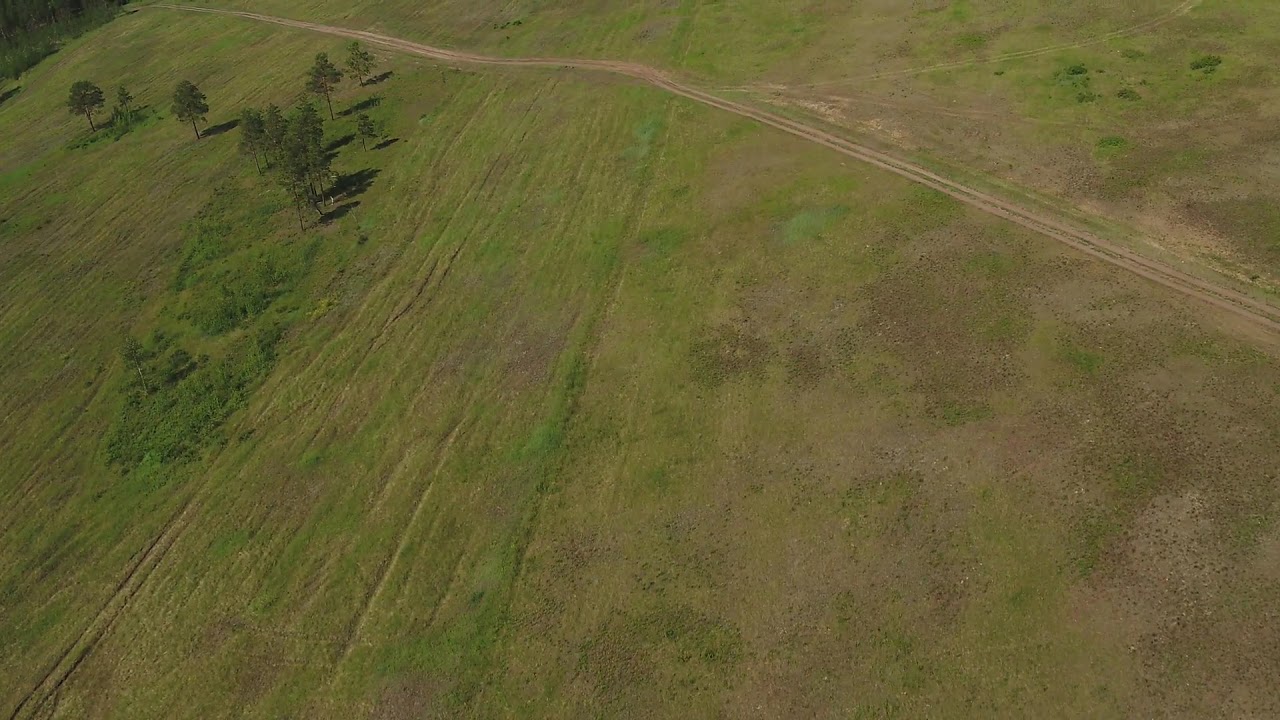This aerial view, likely captured by a drone, showcases a large, grassy field, sparsely dotted with a few medium-sized deciduous trees. The field features a double-track dirt road running diagonally from the middle of the right edge to the top left corner of the image. The landscape includes patches where the grass has worn away to reveal dirt, and there are visible tire ruts particularly on the left side. The left side also contains a small dip in the ground with taller grass and trees that extend slightly beyond this area. There are no buildings, ponds, or other structures visible, and the field appears to be mowed, maintaining relatively low grass without any significant mounds. The image suggests a former farm field or an open plot of land at the edge of a more densely packed forest or grove of trees.